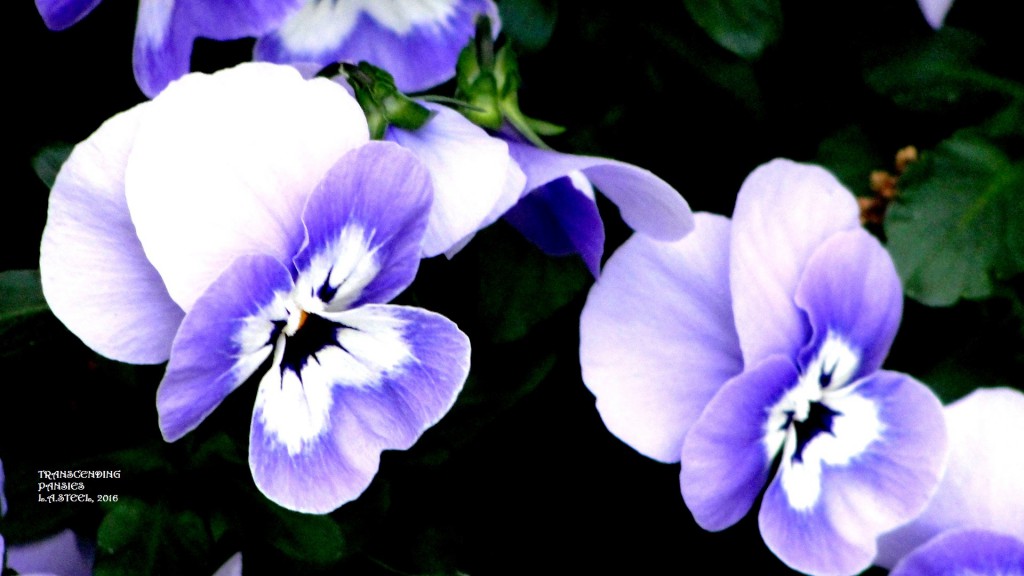The image captures a couple of light purple flowers, possibly pansies, set against a daylight outdoor background of green leaves. The two primary blooms are prominently positioned in the foreground: the larger one on the left occupies almost half of the image, while the smaller one is slightly lower and to the right. Each flower features petals that gradient from light lilac at the edges to white, culminating in dark, almost black centers with tiny yellow dots. In the background, additional flowers and dark green foliage are partially visible, adding depth to the scene. The image is horizontally oriented, longer than it is tall. In the lower left corner, there are three lines of very small white text, possibly a photo credit, though the lettering is too small to discern the details. The overall scene is bright, with a distinct natural light illuminating the flowers and leaves.